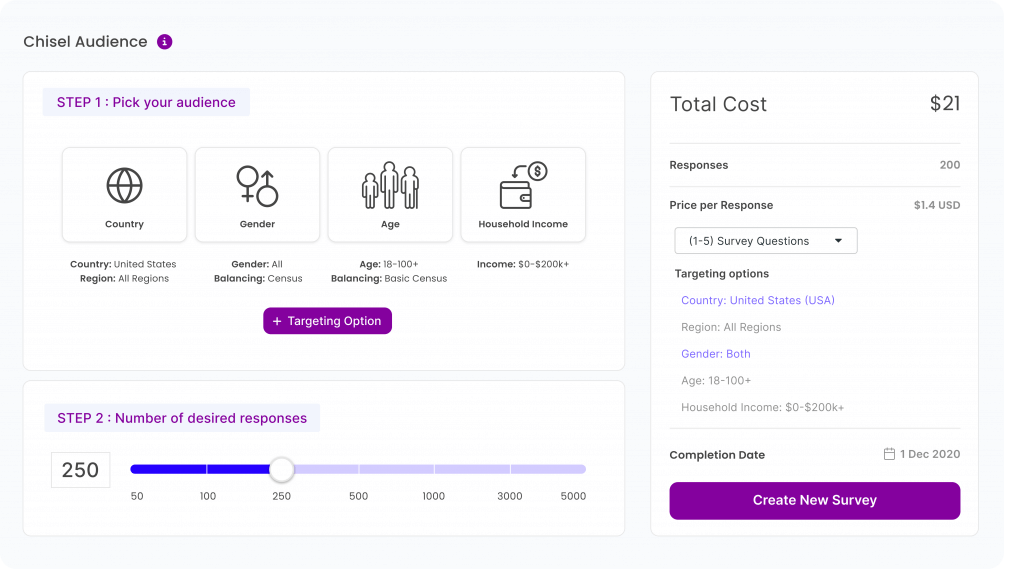The image is a horizontally rectangular screenshot of an order page, set against a very light gray background. In the top left corner, there is a "Chisel Audience" title accompanied by a purple information icon button.

Below this, the page is divided into three distinct sections. The two sections on the left are aligned vertically and are horizontally rectangular, while the section on the right is vertically rectangular.

### Top Left Section:
- **Step One: Pick Your Audience**
  - Several selection boxes for:
    - Country
    - Gender
    - Age
    - Household Income
  - At the bottom center, there is a button labeled "Plus Targeting Option" to add additional targeting options.

### Bottom Left Section:
- **Step Two: Number of Desired Responses**
  - A box on the left displaying the number 250.
  - Adjacent to this box is a slide bar for adjusting the number of desired responses.

### Right Section:
- **Order Summary**
  - **Top Left:** Total cost
  - **Top Right:** $21
  - **Responses:** 200
  - **Price Per Response:** $1.40 USD
  - An expanded dropdown menu showcasing:
    - Survey Questions: 1 through 5
    - Targeting Options:
      - Country: United States
      - Region: All Regions
      - Gender: Both
      - Age: 18 to 100+
      - Household Income: $0 to $200,000
  - **Completion Date:** 1st December 2020
  - At the bottom, there is a purple "Create New Survey" button.

This detailed breakdown captures the essence and layout of the order page, providing a comprehensive and organized overview.